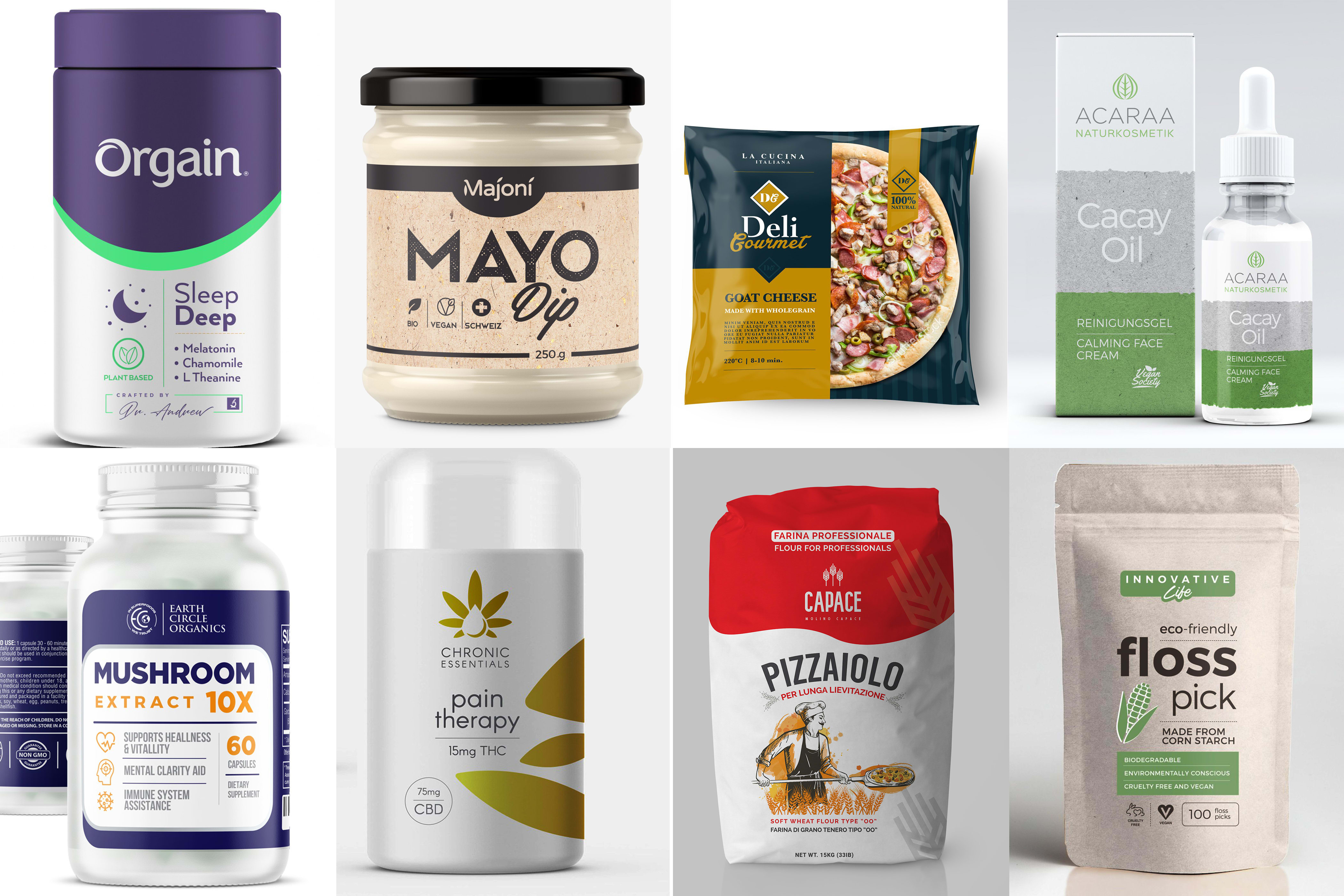The photograph showcases a collection of eight different products arranged in a neatly organized layout, suggesting a storefront or shop page display. In the top left corner sits a cylindrical container labeled "Organe Sleep Deep," adorned with a purple top and a green band. The label details it as a plant-based sleep aid containing melatonin, chamomile, and L-theanine. Moving right, the next item is "Mayo Dip by Mijoni," packaged in a jar. Adjacent to the mayo dip is a "Deli Gourmet Goat Cheese Pizza," clearly marked but with smaller, unreadable text. Continuing to the right is a product titled "Acara Cacay Oil," displayed in a small bottle alongside its packaging.

Transitioning to the bottom row, on the far left is a silver canister labeled "Mushroom Extract 10X" by Earth Circle Organics, purporting to support health, vitality, mental clarity, and the immune system. To its right is a "Chronic Essentials Pain Therapy" product, which contains 50mg THC and 75mg CBD. Next is a package of flour marked "Cappacce Pizziaolo," hinting at its use in pizza making. The final item on the bottom right is an "Innovative Life Eco-Friendly Floss Pick," packaged in a beige, biodegradable paper container. The products are set against a variety of white and grey backgrounds, further enhancing the clean, organized appearance of the display.